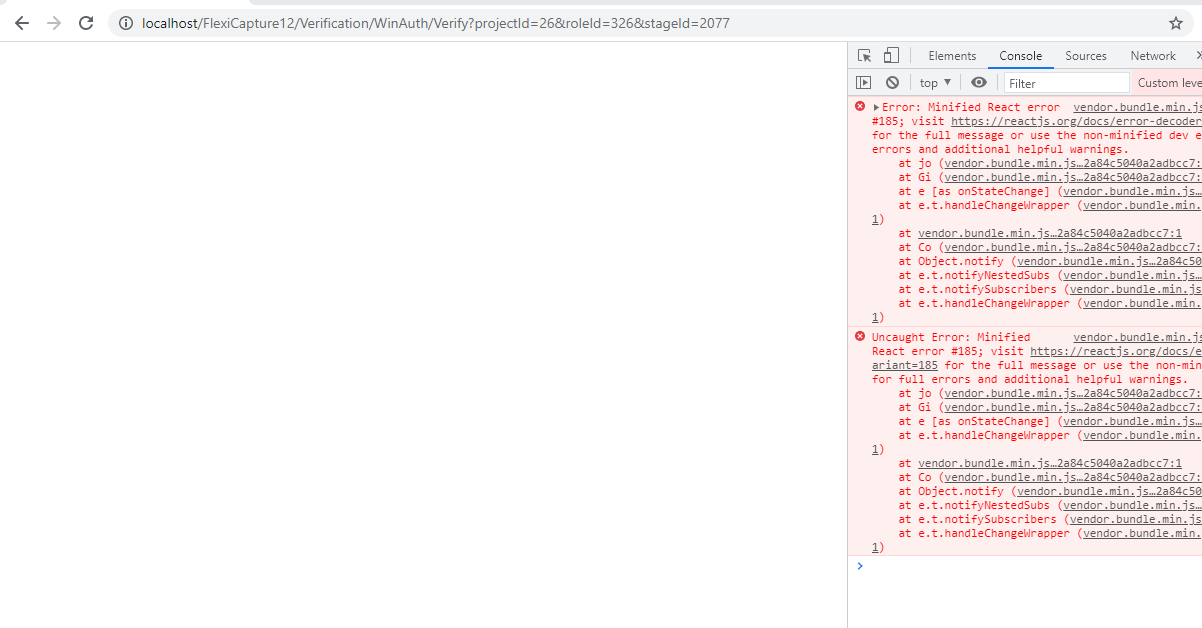This screen capture displays a web interface on a localhost site labeled "FlexiCapture12," followed by a string of letters and numbers. At the top of the interface are gray back and forward navigation arrows, with the forward arrow grayed out, alongside a refresh button shaped like a circle arrow. The browser's search bar features a visible gray star icon, while the primary content area is predominantly white.

On the right side of the image is a section with a light pink background containing detailed error messages. This section includes a mixture of red and black text, links, and several gray UI elements. Notably, there are two gray boxes: one resembling a window with a mouse cursor and another one akin to a document icon.

Below this, a bar labeled "Elements Console" features a thin blue line, with additional tabs such as "Sources" and "Network." Further down, there's a window with a play button, a circle with a slash through it, and a dropdown labeled "top" with an accompanying arrow. Nearby, a gray eye icon and a white filter box are visible with "Custom LEVE" text cut off.

The error message section is characterized by a reddish-pink background, containing multiple red "X" icons next to clickable black links. The errors detail a blend of numbers and letters, presented with red and black fonts. Although smaller, additional red "X" icons and text further down emphasize the detailed nature of the error messages, with no other notable elements in the image.